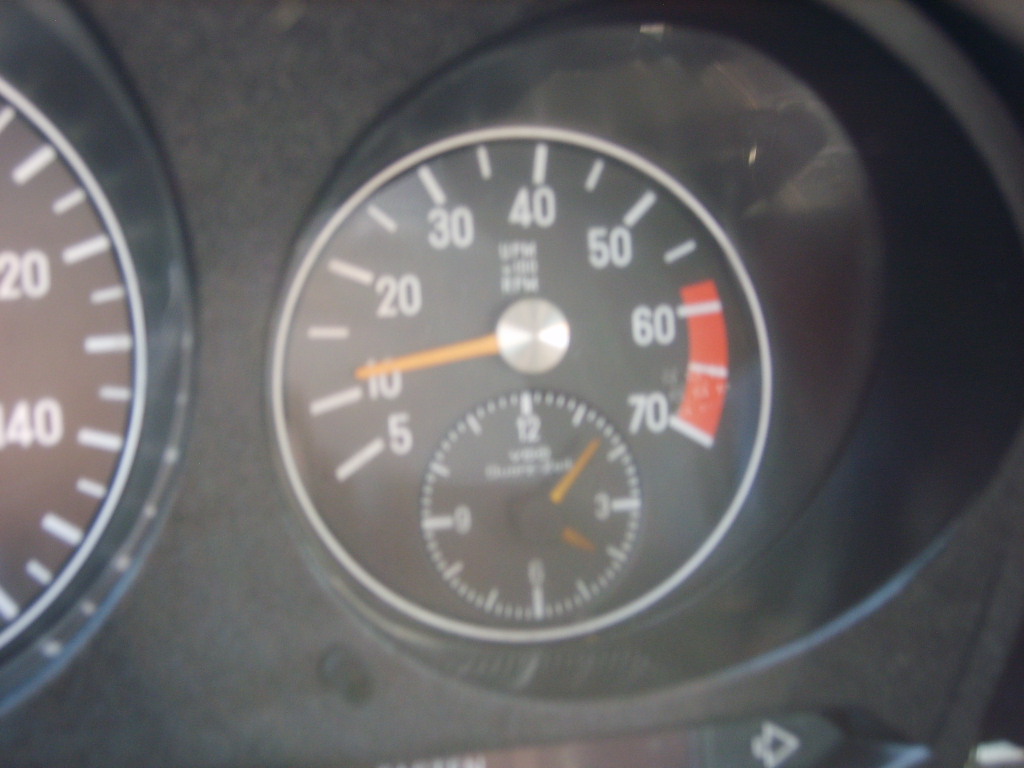A detailed, descriptive caption for the image provided would be:

"An up-close photo focused on a car's speedometer, showcasing the intricate details of the gauge cluster. Central to the image is a circular speedometer with a white background and chrome accents. An orange needle points slightly past the 10 mph mark. The speedometer ticks in increments of 5, 10, with single dashes between major numbers, and extends up to 70 mph, with the area between 60 and 70 highlighted in red to indicate the redline zone. To the left, a partial view of another gauge is visible, displaying a white circular face with dashes and numbers, but only a segment is seen. Embedded below the main speedometer is a classic-style clock, featuring a black center and two orange hands, indicating the time as 4:07."